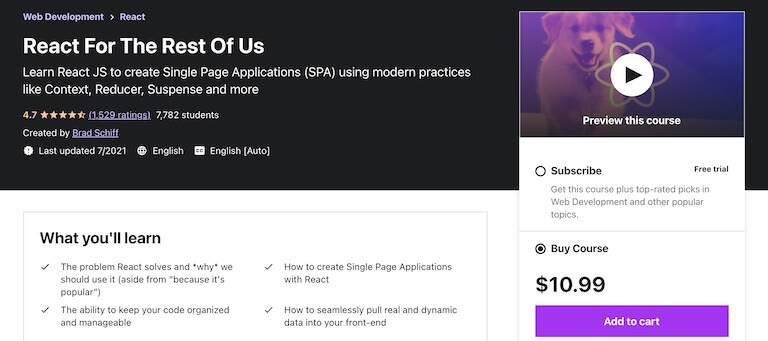A detailed description of a screenshot of an online course purchase page.

---

The screenshot showcases a computer monitor, likely a laptop or desktop, displaying a webpage that resembles an online course purchase page. The course in question is titled "React for the Rest of Us," and it falls under the Web Development category, as indicated in the top left-hand corner.

The visual layout of the webpage is split horizontally. The upper half features a black banner with white text, while the lower portion presents black text on a white background. On the right side of the screen, there's an embedded image of a dog with an interactable play button overlay labeled "Preview this course."

Beneath this, the purchase options are displayed with two choices. The first option allows users to subscribe for a free trial, featuring a selectable circle. Once selected, the circle fills in. The text accompanying this option reads "Get this course plus top-rated picks in web development and other popular topics."

The second option, labeled "$10.99," is pre-selected. This selection also includes a circle that fills in when chosen, accompanied by the label "Buy course." Directly below these options is an interactable "Add to Cart" button.

Further down, a section titled "What You'll Learn" details the course's coverage. It explains that the course addresses the problem React solves, the reasons to use React beyond its popularity, methods for maintaining organized and manageable code, techniques for creating single-page applications with React, and the process of integrating real and dynamic data into the front end.